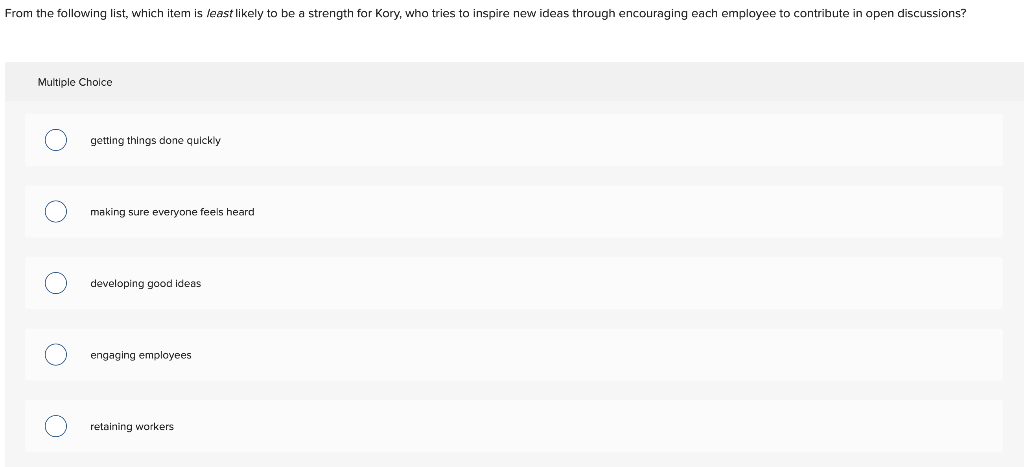The image features a clean white background with black text at the top, posing the question: "From the following list, which item is least likely to be a strength for Corey, who tries to inspire new ideas through encouraging each employee to contribute in open discussions?" Beneath this text, there is a multiple-choice section with a gray background and black text. To the left, it says "Multiple Choice," followed by five options, each accompanied by a blank selection button. The options are: "Getting things done quickly," "Making sure everyone feels heard," "Developing good ideas," "Engaging employees," and "Retaining workers." None of the selection buttons are marked.